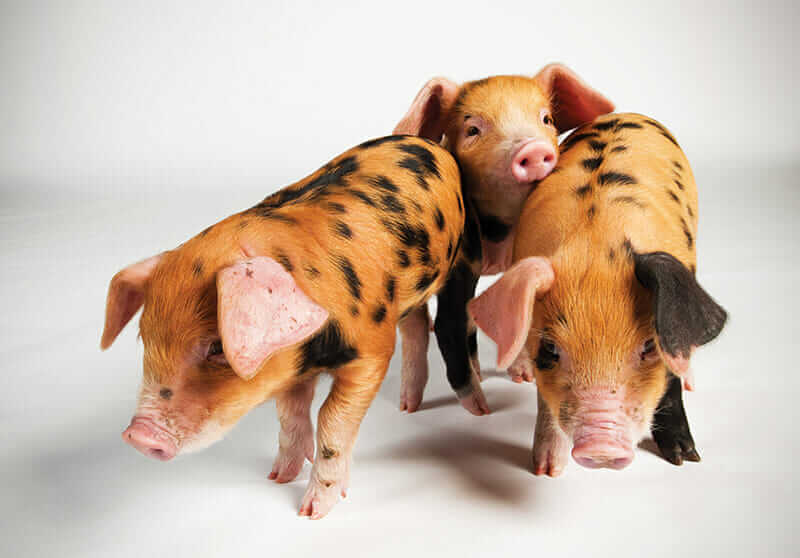This photograph captures three adorable piglets against a white background. In the foreground, two piglets stand side by side displaying their unique fur patterns — a rusty orange color adorned with varying black and brown spots, much like those you'd see on a dog or cat. The piglet on the left foreground showcases pink floppy ears and a combination of pink and black legs, while the one on the right foreground sports one pink and one black ear. Both have characteristic pink snouts and little pig's feet. The third piglet, smaller in size, is positioned in the background with his nose comfortably resting on the back of the right foreground piglet, presenting an endearing scene of camaraderie. His large, floppy pink ears add to the charm. Their shadows are subtly cast on the white canvas, highlighting their presence and bringing depth to the image. The innocent, inquisitive faces and the natural posing of these piglets make this photograph irresistibly cute and heartwarming.